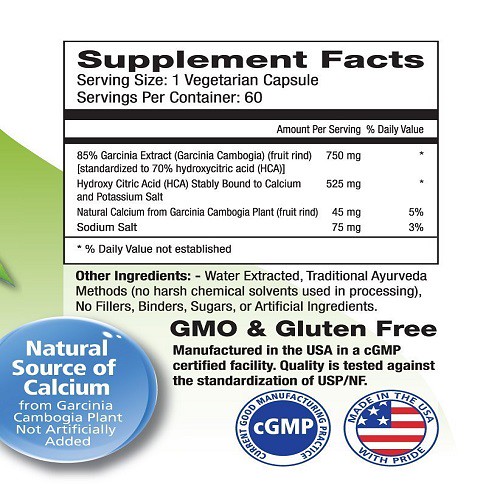The image is of a detailed supplement label for a vegetarian capsule. The label prominently features "Supplement Facts" and specifies a serving size of one vegetarian capsule, with 60 servings per container. Key ingredients are listed in black font, including 750 mg of Garcinia cambogia extract, standardized to 70% hydroxy citric acid (HCA), with components such as 525 mg bound to calcium and potassium salt, 45 mg of natural calcium derived from the Garcinia cambogia plant, and 75 mg of sodium salt. Additional detailed information includes a list of other ingredients, which notably excludes fillers, binders, distributors, or artificial agents, and mentions the use of traditional arubia methods without harsh chemicals or solvents. The product is labeled as GMO and gluten-free, manufactured in the USA in a CGMP certified facility, and tested for quality against USP/NF standards. It also features a circular icon with the American flag, stating "made in the USA with pride," and highlights in blue and white that it’s a natural source of calcium. On the left side of the label, a small section is green, standing out against the predominantly white background.